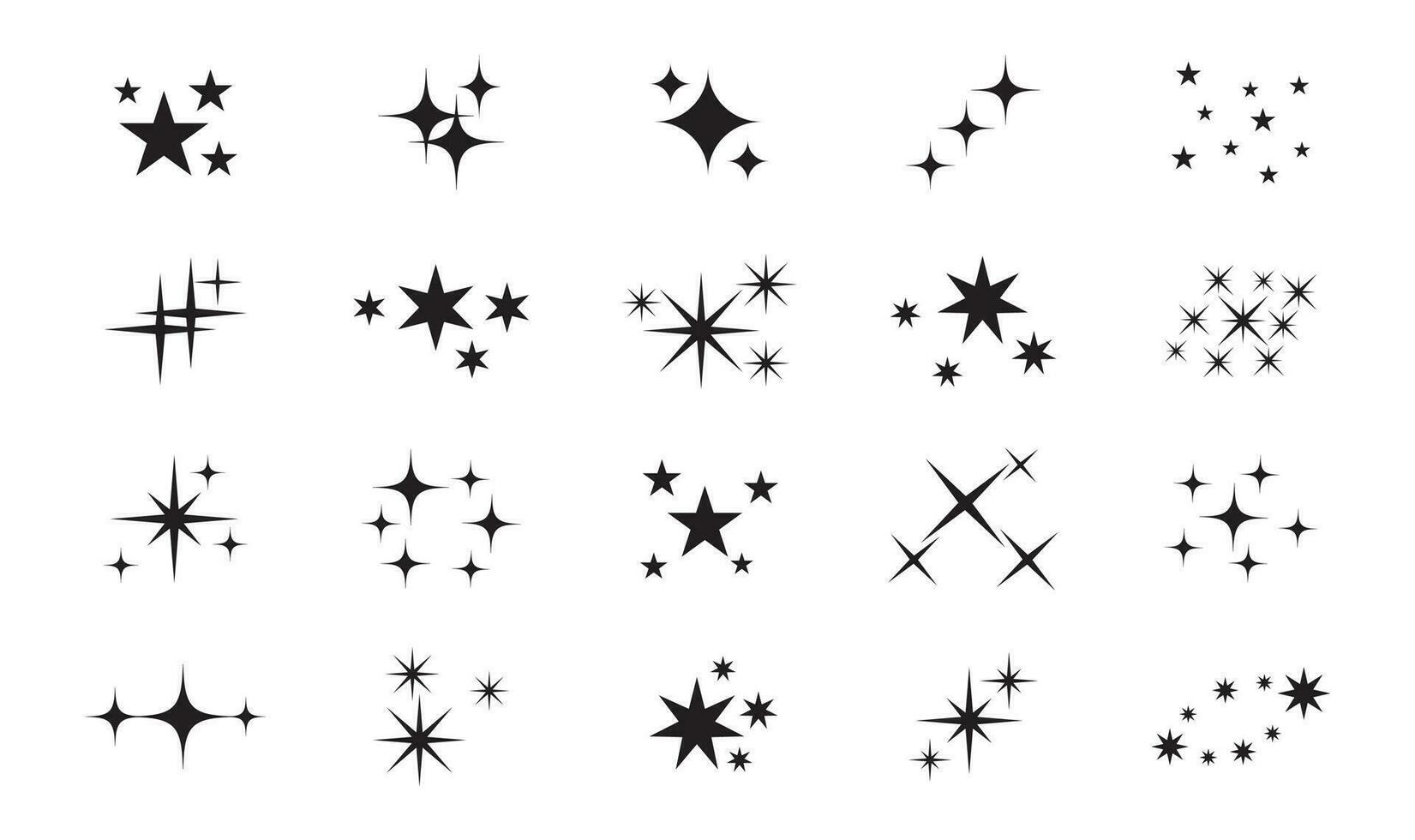This is a detailed illustration showing a 4x5 grid of star-themed graphic images, amounting to a total of 20 distinct designs. Each design varies in shape, size, and composition while maintaining a consistent black color against a stark white background. In the top left corner, one image features a large five-pointed star surrounded by three smaller stars in the top right, top left, and bottom right corners. Adjacent to it, another image displays a four-pointed star with a larger star at the back on the right side. Further along, a graphic consists of a large star with two diminutive stars positioned at the top left and bottom right corners. Another design showcases three stars progressively increasing in size from the bottom lower right corner upwards. Additionally, some images depict intricate clusters, such as three larger stars encircling six smaller ones. Each row contains five unique clusters of stars, arranged into four rows total, ultimately forming a visually striking and diverse collection of stylized star graphics that range from simple, straight-line designs to more complex and ornate configurations. These stars are not realistic depictions of celestial stars but stylized renditions drawn for graphical representation.